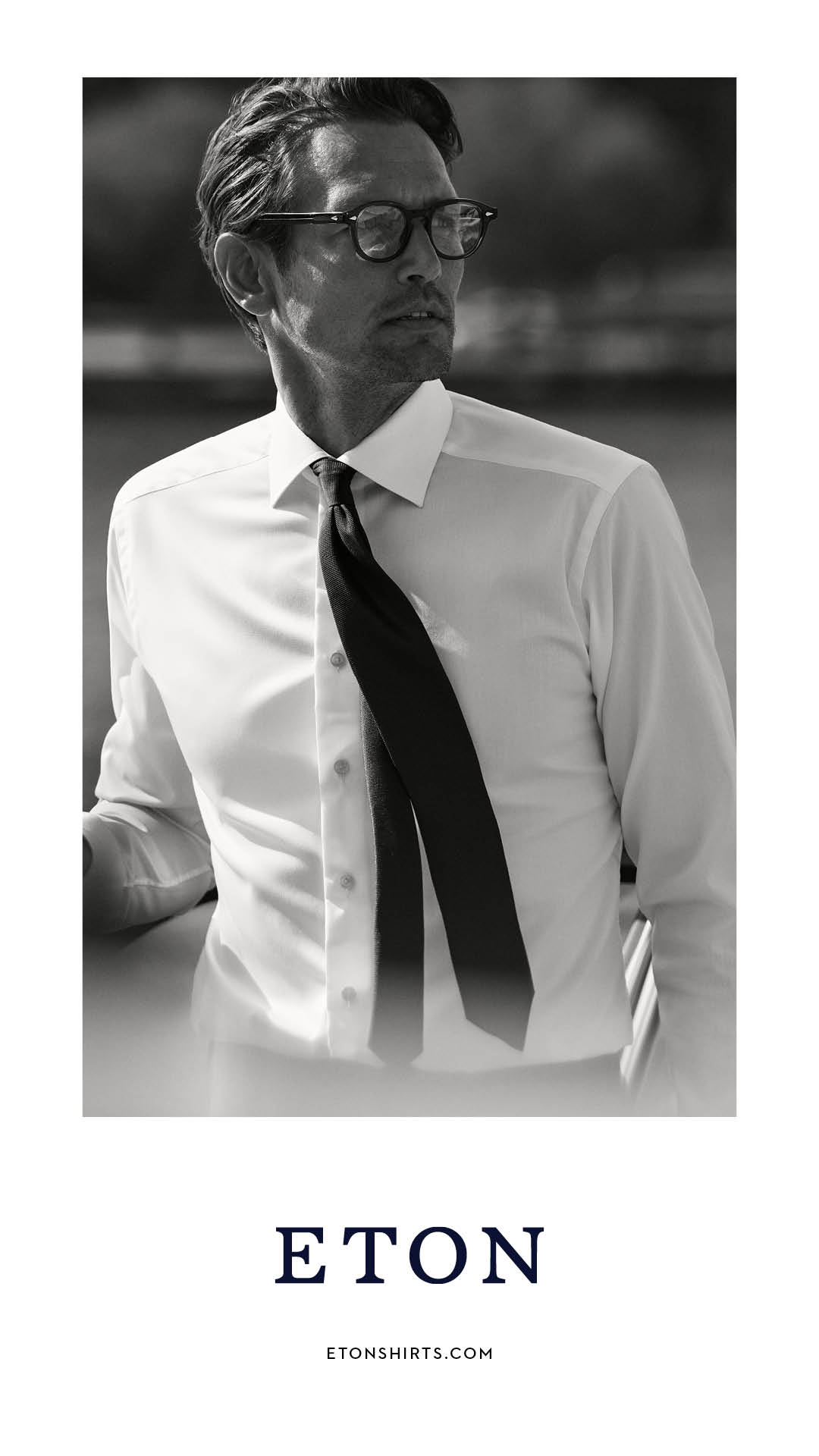This black-and-white advertisement features a sharply dressed male model donning a fitted white button-up collared shirt paired with a black tie that appears to be caught in the wind, swinging towards the left side of his body. He sports thin-rimmed glasses, has short hair, and a partial mustache, adding to his meticulously groomed appearance. The man is captured from the waist up, facing sideways while walking forward, seemingly intrigued and focused on something off to his shoulder. The blurred background ensures he remains the focal point of the image. At the bottom of the image, bold text reads "E.T.O.N." with smaller text underneath stating "EtonShirts.com," indicating it is an advertisement for Eton Shirts.